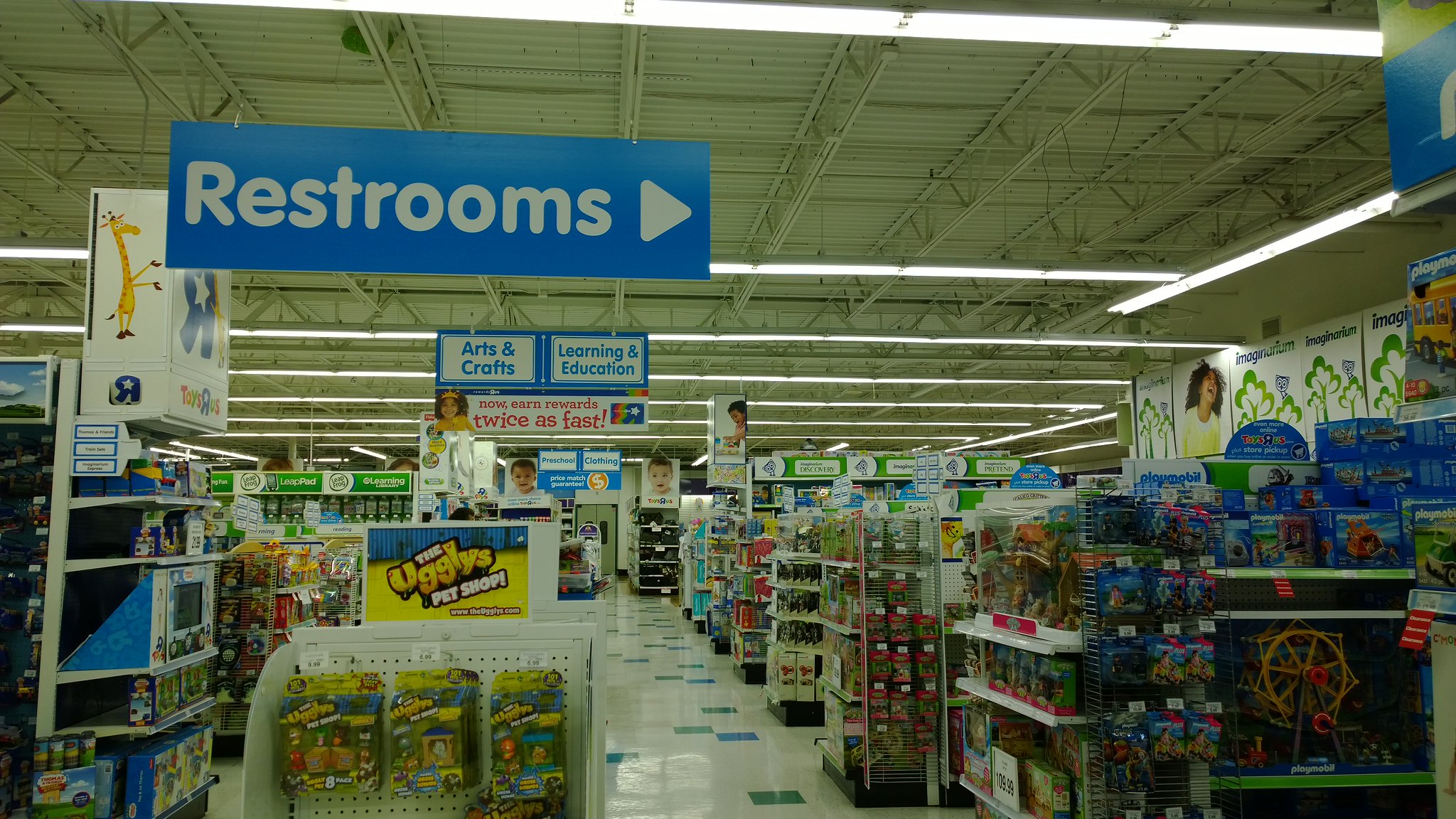The image captures the interior of a large Toys R Us store with an open ceiling, exposing metal rafters and numerous hanging fluorescent lights that illuminate the space. Dominating the upper section of the frame is a prominent blue rectangular sign with white text that reads "Restrooms," accompanied by an arrow pointing to the right. Directly behind this sign is a larger white sign displaying a graphic of a giraffe and the familiar Toys R Us logo, reinforcing the store's identity. The store's floor consists of white tiles interspersed with random blue and green tiles. The perspective of the image is down a central aisle, flanked by several horizontal aisles filled with various toys on shelves. In the bottom right-hand corner, a Ferris wheel toy is distinctly visible, adding a playful element to the scene.